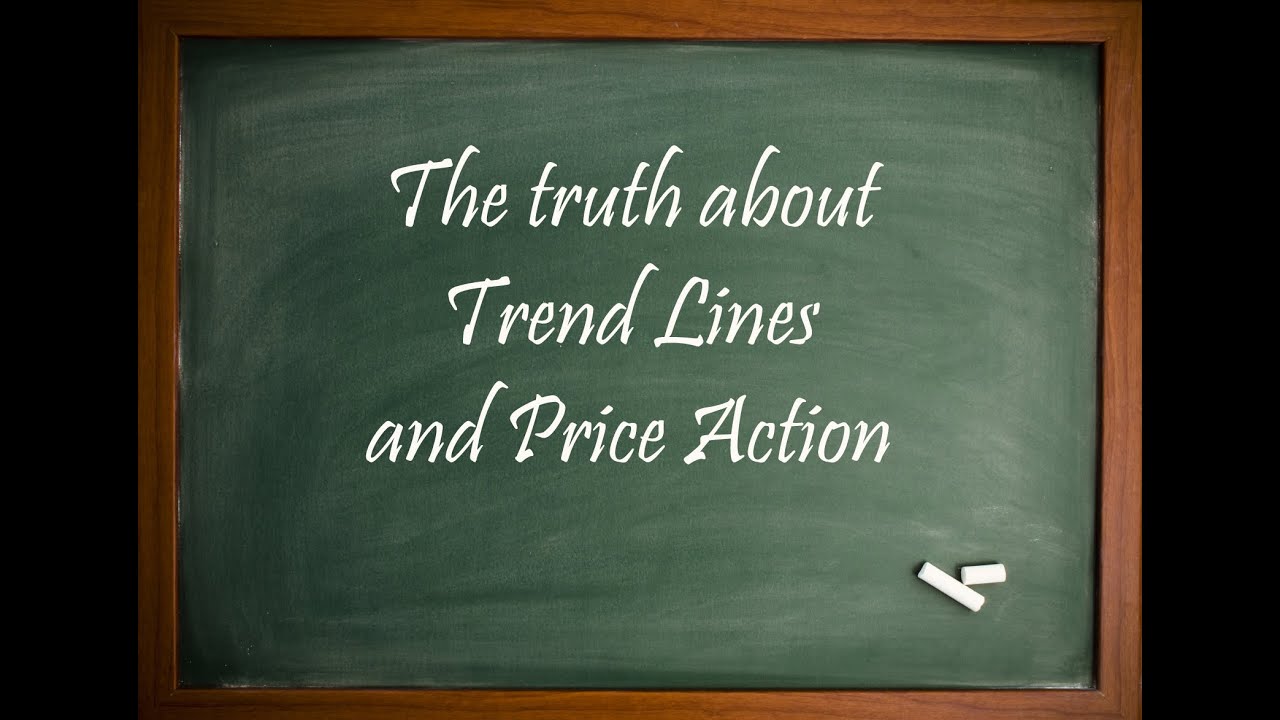The image displays a traditional green chalkboard with a slender wooden frame, centered against a black backdrop. The chalkboard has a rectangular shape, with its width being longer than its height. Written on the chalkboard in elegant, slightly slanted cursive-like font are the words: "The truth about trend lines and price action." In the bottom right corner, there are two pieces of white chalk; one intact and one broken, positioned in a crisscross pattern. The meticulous arrangement of the chalk suggests a deliberate design choice. The overall scene evokes a classic, academic atmosphere with a modern twist in the sophisticated script of the text.